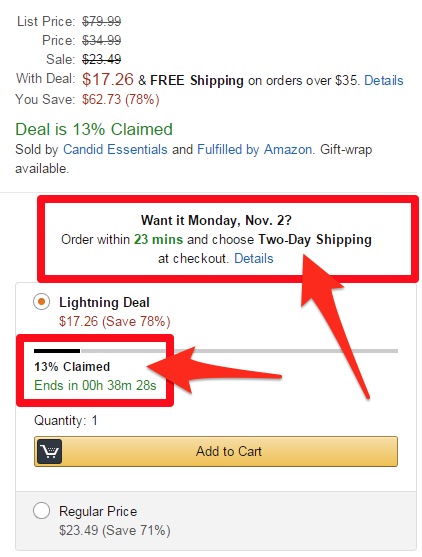The graphic displays a detailed view of a shopping page with numerous discounts and promotional offers. 

At the top, the original list price of $79.99 is shown, but it is struck through. Beneath that, a price of $34.99, also struck through, appears. Following that, a sale price of $23.49, again struck through, is listed. Finally, it reveals the current deal price of $17.26 highlighted in red, accompanied by "free shipping on orders over $35.00."

Additionally, there's a note in red: "You save $62.73 (78%)." Below this, the status indicates that 13% of the deal has been claimed. The product is sold by Candid Essentials and fulfilled by Amazon, with an option for gift wrapping.

A red rectangle with an arrow pointing to it advises, "Get it by Monday, November 2nd," if ordered within 23 minutes and choosing 2-day shipping at checkout. This is marked as a "Lightning Deal" with the deal price of $17.26 in red, reiterating the 78% savings.

Further down, another red rectangle with an arrow shows that the deal is 13% claimed, ending in 00H38M28S. The available quantity is noted as "1."

There is a prominent yellow "Add to Cart" button, with an unchecked or unfilled button below that reiterates the regular price of $23.49 alongside a 71% savings message in parentheses.